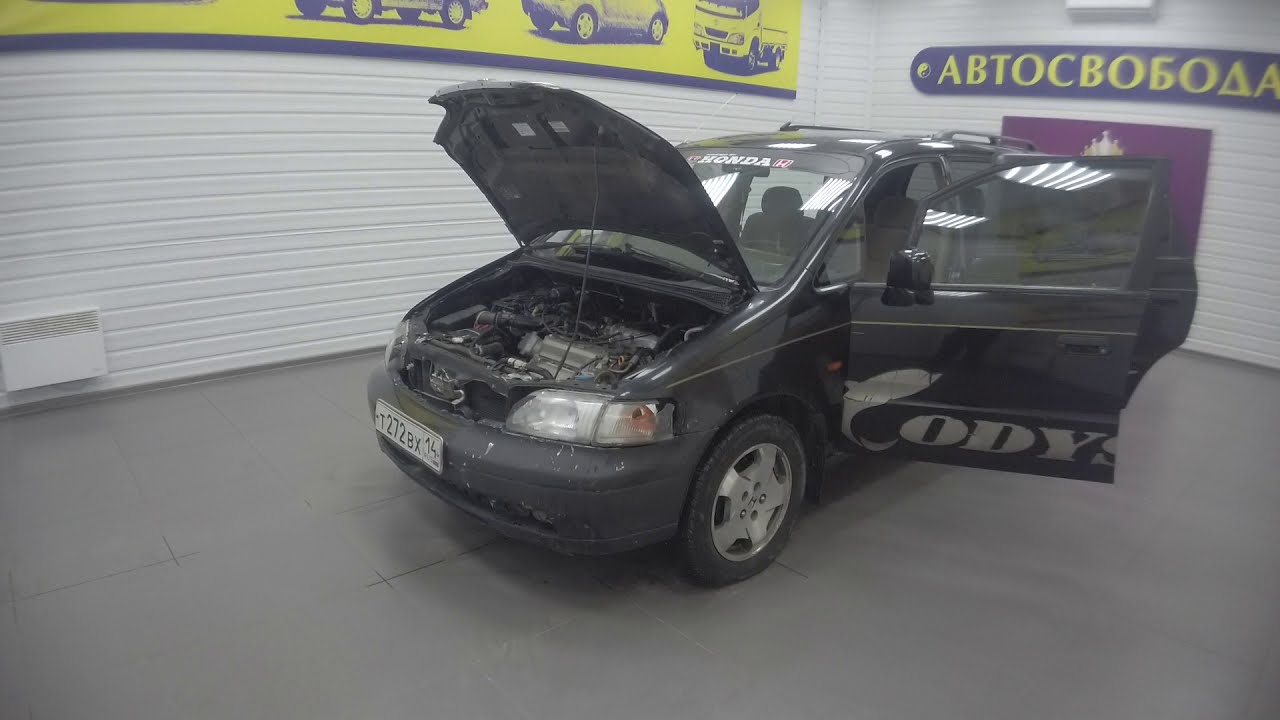This detailed indoor photograph, likely taken in a garage or body shop under fluorescent lighting, features a black Honda van or SUV prominently displayed with its hood up, revealing a silver and black engine, and all its doors open. The vehicle, which has the word "Honda" emblazoned in white across the top of the windshield alongside the red and white Honda symbol, rests on a plain gray floor. The front driver's side door displays the name "Cody" in white lettering near the bottom. The room has white wood-paneled walls with a few distinct decorations: on the left-hand wall, there is a stylized yellow and blue image of several partially obscured cars, likely including a box truck, while on the back right-hand wall, a blue plaque with yellow Greek or Russian letters and a yin-yang symbol is visible. Additionally, the white brick walls feature a white vent, contributing to the utilitarian atmosphere of the space. The entire setting underscores the focus on the van, highlighting its open state from various detailed angles.